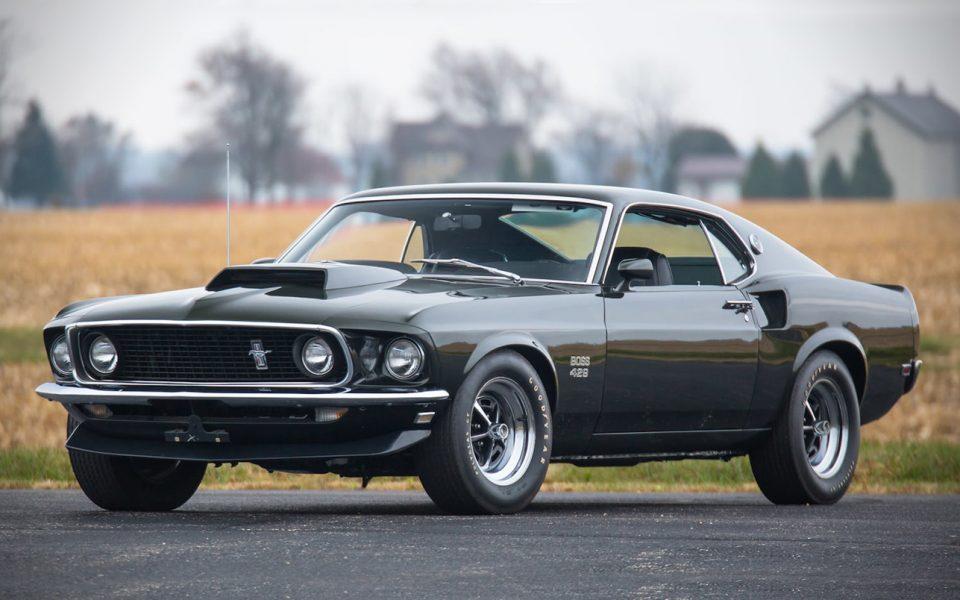The image depicts a pristine, black vintage 1969 Boss 428 Mustang. The car is parked on a gray asphalt road and faces to the left, showcasing its aggressive stance. It features four round headlights at the front, two integrated into the grille which proudly displays the iconic Mustang pony emblem. A prominent hood scoop and "Boss 428" text on the fender emphasize its powerful nature. The car sports chrome rims and Goodyear tires with white lettering, all in impeccable condition. The windshield and other trim elements are lined with silver. The background reveals a blurred, brownish field, possibly a cut-down cornfield or one with dead grass, with some trees and houses partially visible under a gray, hazy sky. The striking details and clean finish of the Mustang make it the focal point of the composition.